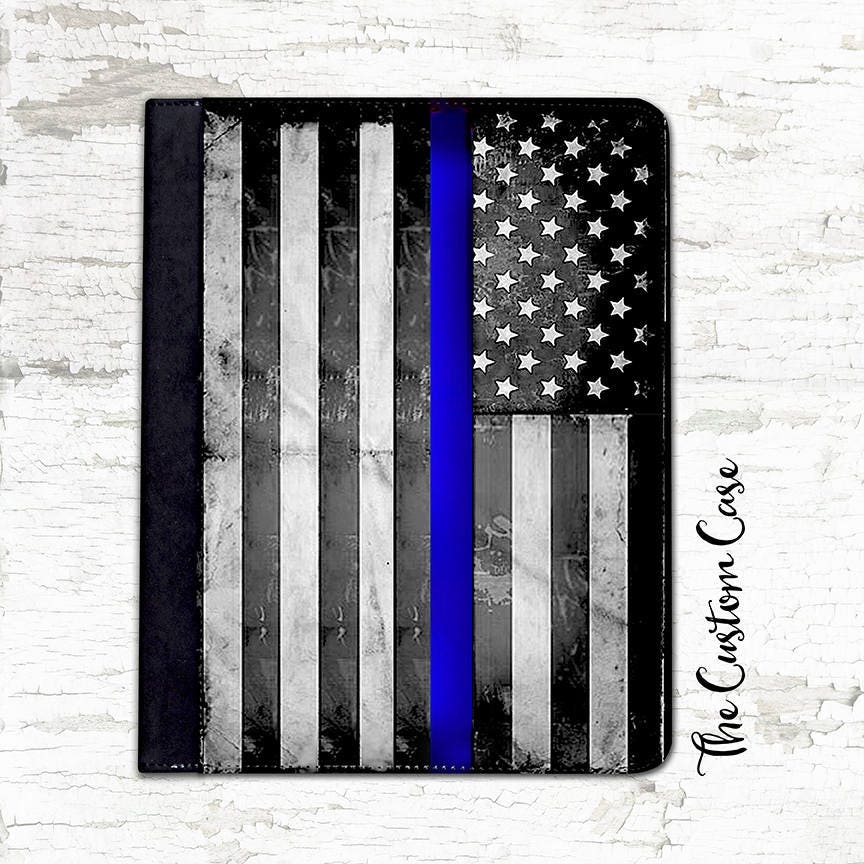The image showcases a perfectly square photograph with a backdrop resembling a whitewashed wooden surface, where chipped paint reveals gray wood underneath. At the center of the image is a rectangular item in portrait orientation, appearing to be an iPad or binder case, with slightly rounded top and bottom right corners while the left corners remain squared. This case mimics an American flag turned sideways, featuring black and white stripes with a standout bright blue stripe running vertically. The top right-hand corner of the case presents a black field adorned with white stars. It’s evident that the case, with visible stitching and a worn, dirty appearance, has been well-used. Written in cursive near the right side of the case is the phrase "the custom case."